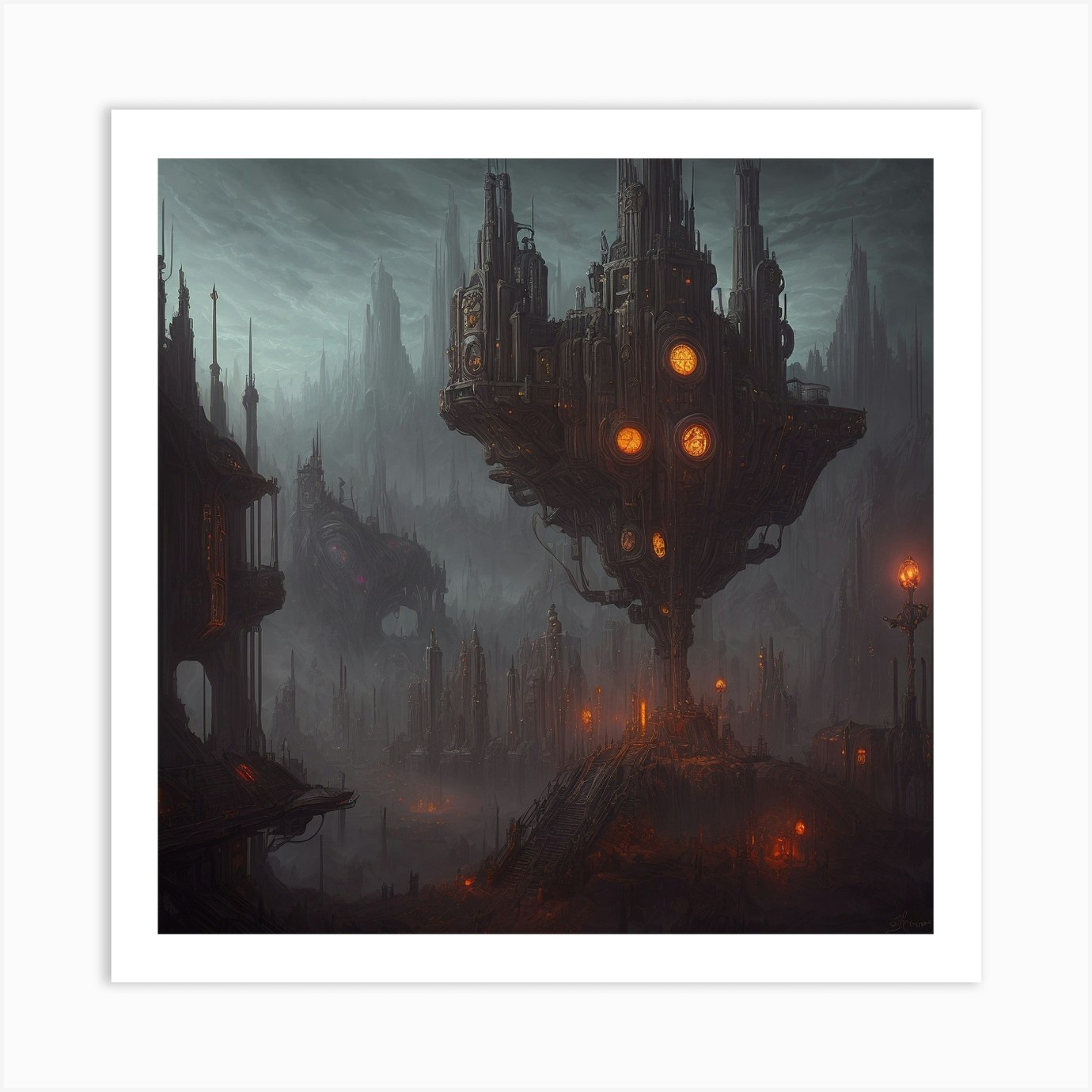The image depicts a dark, dystopian landscape with a dense, foggy, nighttime sky shrouded in deep greys and blacks. The lower part of the picture features a foggy, dark terrain interspersed with streaks of orange light emanating from various sources, possibly light poles. Prominently in the lower right corner, a craggy pile of rocks rises, from which a tree trunk-like structure emerges. This tree trunk has branches extending to the left and right, and about a third of the way up, a massive building, possibly a castle, is perched atop it. The building is characterized by multiple levels, towers, and spires that stretch into the sky, some of which have antennas. This structure's facade is adorned with round features resembling clocks or stained glass windows in orange hues. The background shows shadowy, pointy skyscrapers that resemble jagged rocks jutting upwards, contributing to the eerie and desolate atmosphere. The composition, bordered by a white frame, looks like it could be a computer-generated animation of an alien planet or a dystopian future, with an overall creepy and unsettling ambiance.